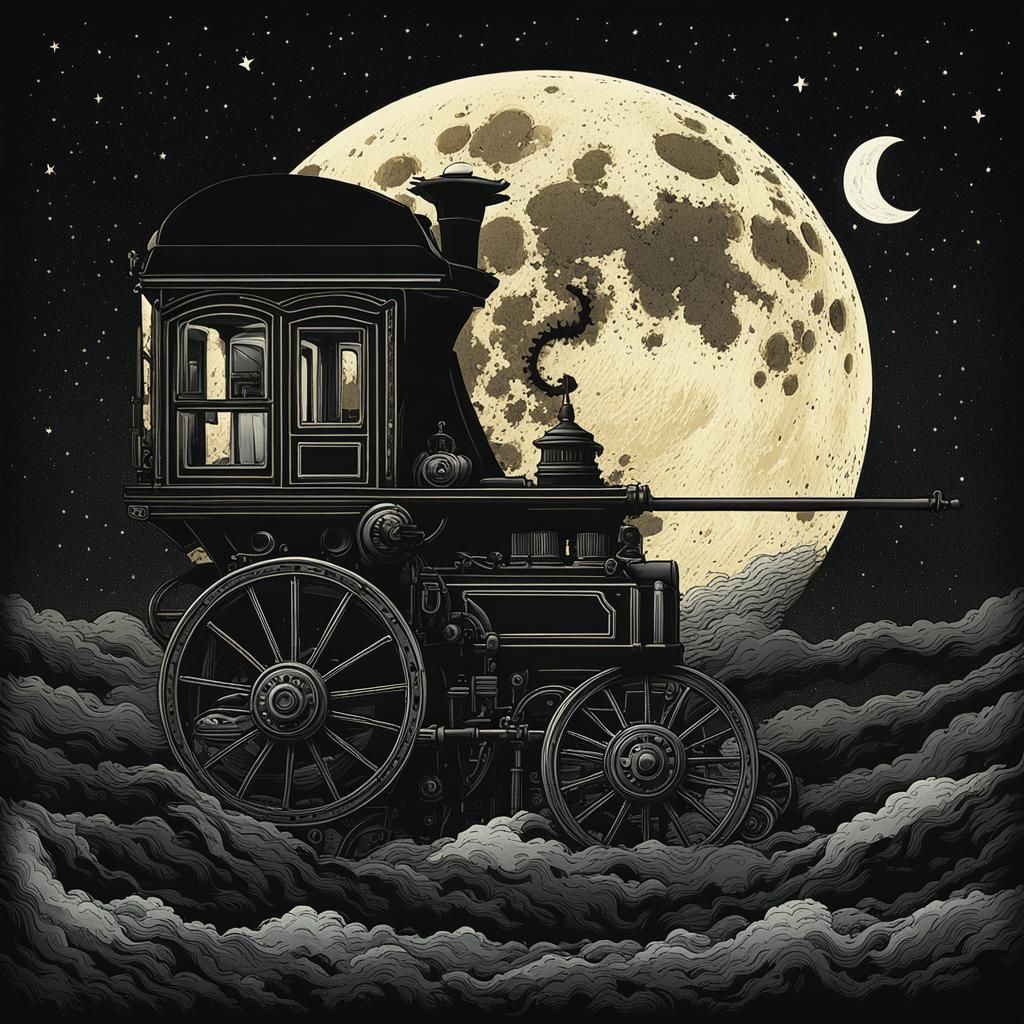This detailed artwork presents a steampunk-inspired scene set in a surreal night sky. Dominating the top half of the image is a grand, luminous full moon, intricately textured with white and black spots. In the upper right corner, a smaller crescent moon adds a whimsical touch. The backdrop features an array of twinkling stars, enhancing the celestial ambiance. The bottom half is shrouded in dense, swirling clouds rendered in shades of gray, black, and charcoal. At the center of the composition, partially obscuring the moon, is a vintage black carriage-like vehicle with prominent silver wheels. This steampunk train, exuding an old-world charm, appears to be gliding through the clouds, or possibly enshrouded in smoke from its own movement. The vehicle, with its long pole protruding from the front and suggested windows at the rear, is meticulously designed, making it the focal point of this captivating, dreamlike cartoon imagery.